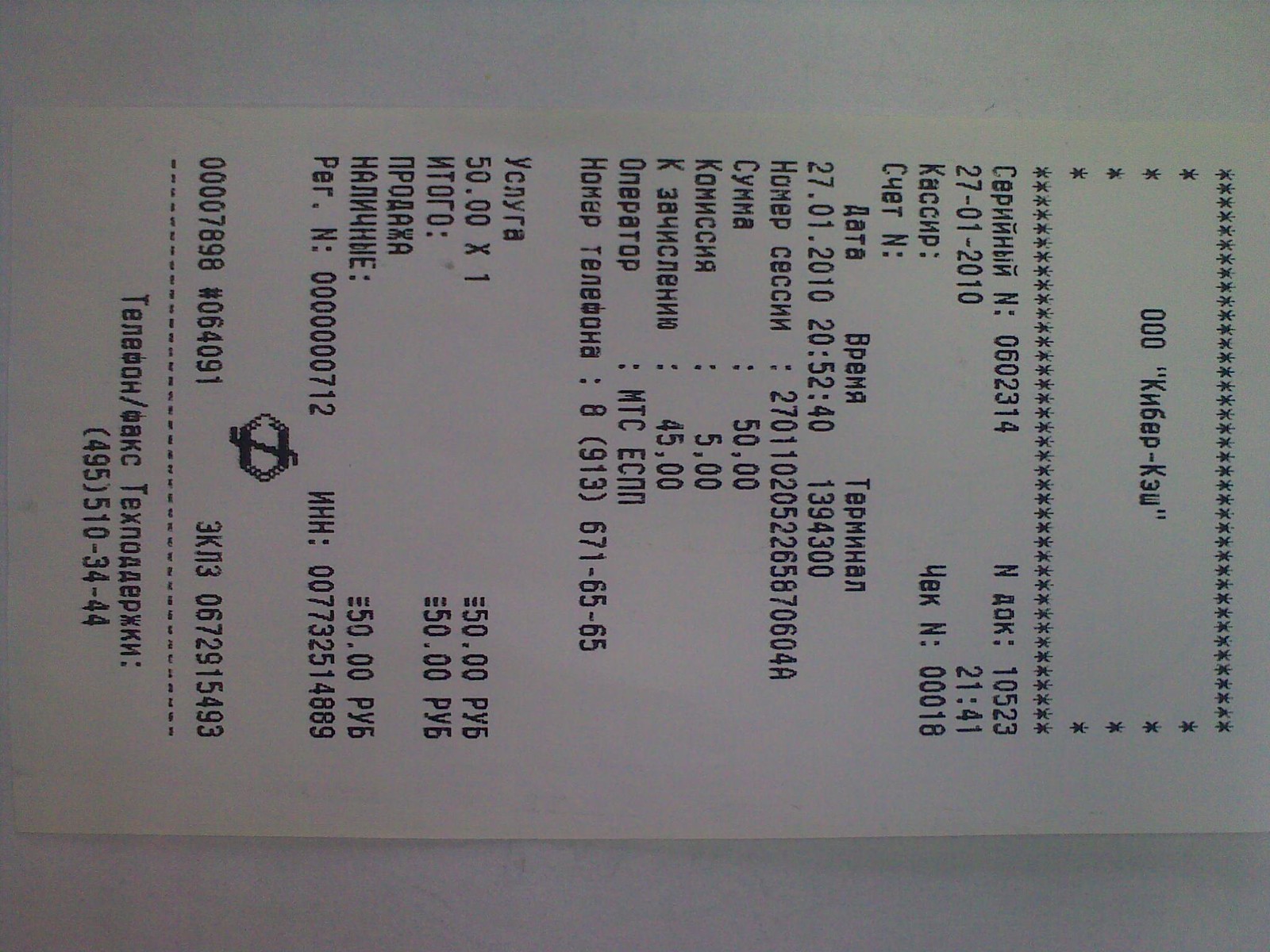This detailed image shows a white receipt with black writing, primarily in Russian, possibly from a cash register. The receipt is oriented sideways to the right. At the top of the receipt, a box made of stars encloses the number "000". Below this, there is a date indicating January 27th, 2010 (27-1-2010), and a timestamp of 21:41. Various charges are listed, including amounts of $50, $5, and $45. Towards the bottom of the receipt, a phone number (495-510-3444) is visible along with additional numbers and text in Russian.